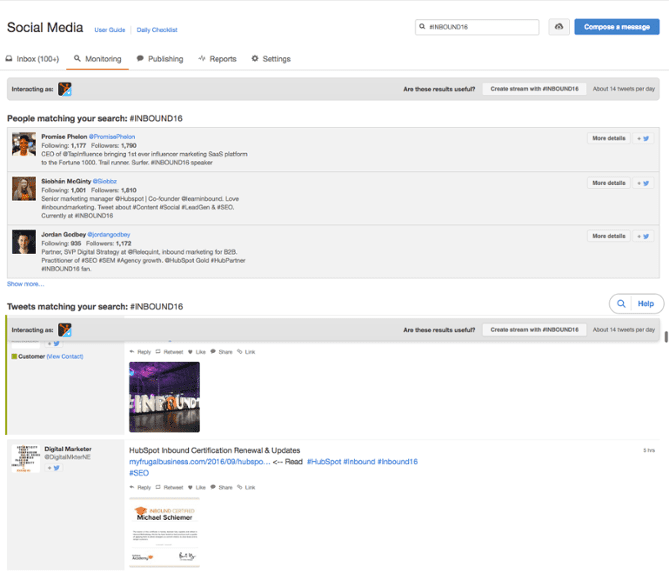This screenshot showcases the interface of a website or software application titled "Social Media," prominently displayed in the top left corner. Adjacent to the title are hyperlinks directing users to a user guide and a daily checklist. Dominating the right-hand side of the header is a search box, accompanied by a blue button labeled "Compose a Message."

Below the header, a series of navigational buttons offer options to filter content, including "Inbox," "Monitoring," "Publishing," "Reports," and "Settings." This platform appears to facilitate searching for hashtags on social media.

In this particular instance, the hashtag "nbound16" has been searched. The results include three user profiles matching this hashtag, along with a list of tweets related to "nbound16." The tweets are displayed in a sequential, list format, allowing users to easily peruse the relevant social media activity.

Overall, the screenshot provides a comprehensive view of a social media management tool, highlighting its capabilities for hashtag searches and user interactions.